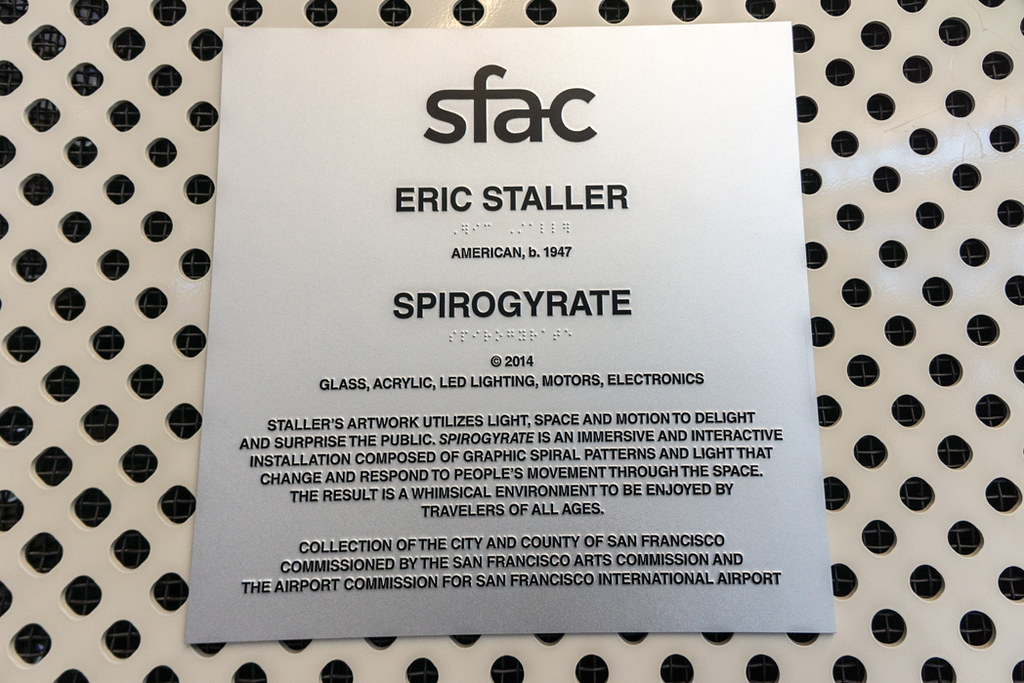This image shows a silver, square-shaped plaque against a polka-dotted background of black and white circles. The plaque prominently features the heading "SFAC," followed by "Eric Stahler" in bold, black, sans-serif text, with corresponding braille text beneath. Below, it reads "American B 1947" and then "Spiralgyrate," also with accompanying braille. Further down, a detailed description explains: "Copyright 2014. Glass, acrylic, LED lighting, motors, electronics. Stahler's artwork utilizes light, space, and motion to delight and surprise the public. Spiral gyrate is an immersive and interactive installation composed of graphic spiral patterns and lights that change and respond to people's movements through the space. The result is a whimsical environment to be enjoyed by travelers of all ages." This piece is part of the City and County of San Francisco collection, commissioned by the San Francisco Arts Commission and the Airport Commission for San Francisco International Airport.